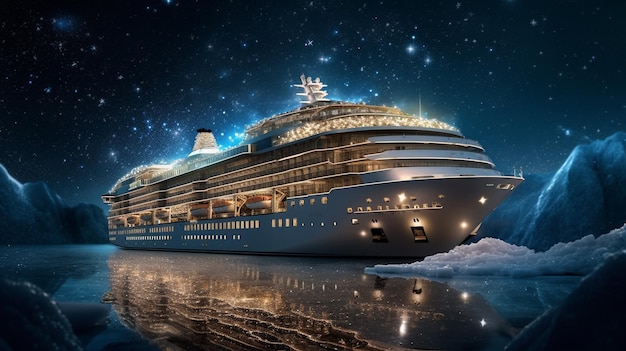In this detailed and hyper-realistic AI-generated illustration, we see a massive white cruise liner navigating icy waters at night. The ship is luminously lit with golden lights, illuminating its multiple decks and reflecting beautifully in the calm water below. The night sky is a dark blue, speckled with countless white and bluish stars. The cruise ship, possibly up to eight levels tall, features numerous windows and lifeboats, alongside a brightly lit smokestack and antenna array, giving it a festive, almost Christmas-like appearance. It sails amidst a treacherous Arctic sea, surrounded by variously shaped and sized icebergs and glaciers. Directly in its path looms a sizable glacier, suggesting that the ship might be in danger. The setting is serene yet desolate, with icy cliffs and snowy mountains encircling the vessel, adding to the sense of isolation and potential peril. The overall scene vividly portrays a grand, glowing ship in a stark, icy wilderness under a star-studded sky.